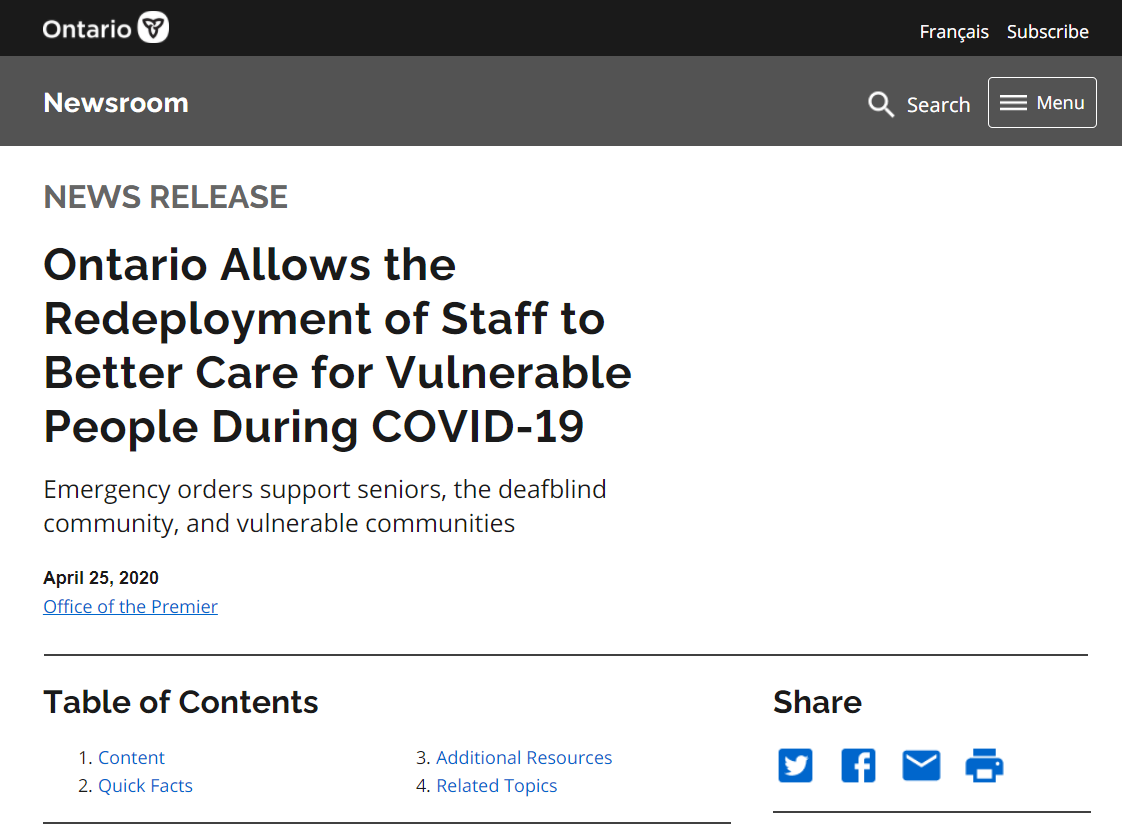This image is a detailed screenshot of a governmental website. At the very top, a black navigation bar features white text, starting with "Ontario" on the left, followed by a white circle with a central logo outlined in black. On the right side of the black bar, the text reads "FRANÇAIS" and "Subscribe." Below, a grey bar presents "Newsroom" on the left and a search icon followed by a menu box on the right.

Further down, the main section begins with grey text reading "News Release" on the left. Directly underneath this, prominent black text announces, "Ontario allows the redeployment of staff to better care for vulnerable people during COVID-19." In smaller lettering below, additional context reads, "Emergency order supports seniors, the deaf-blind community, and vulnerable communities."

Continuing downward, the content is dated "April 25th, 2020" and attributed to the "Office of the Premier." Below this, a text box lists the table of contents which includes: 
1. Content
2. Quick Facts
3. Additional Resources
4. Related Topics

On the right-hand side, there is a "Share" section with several icons: a blue circle with a white bird (Twitter), a blue circle with a white "F" (Facebook), an envelope icon (email), and a printer icon. This section is underlined with a black line delineating the end of this area on the website.